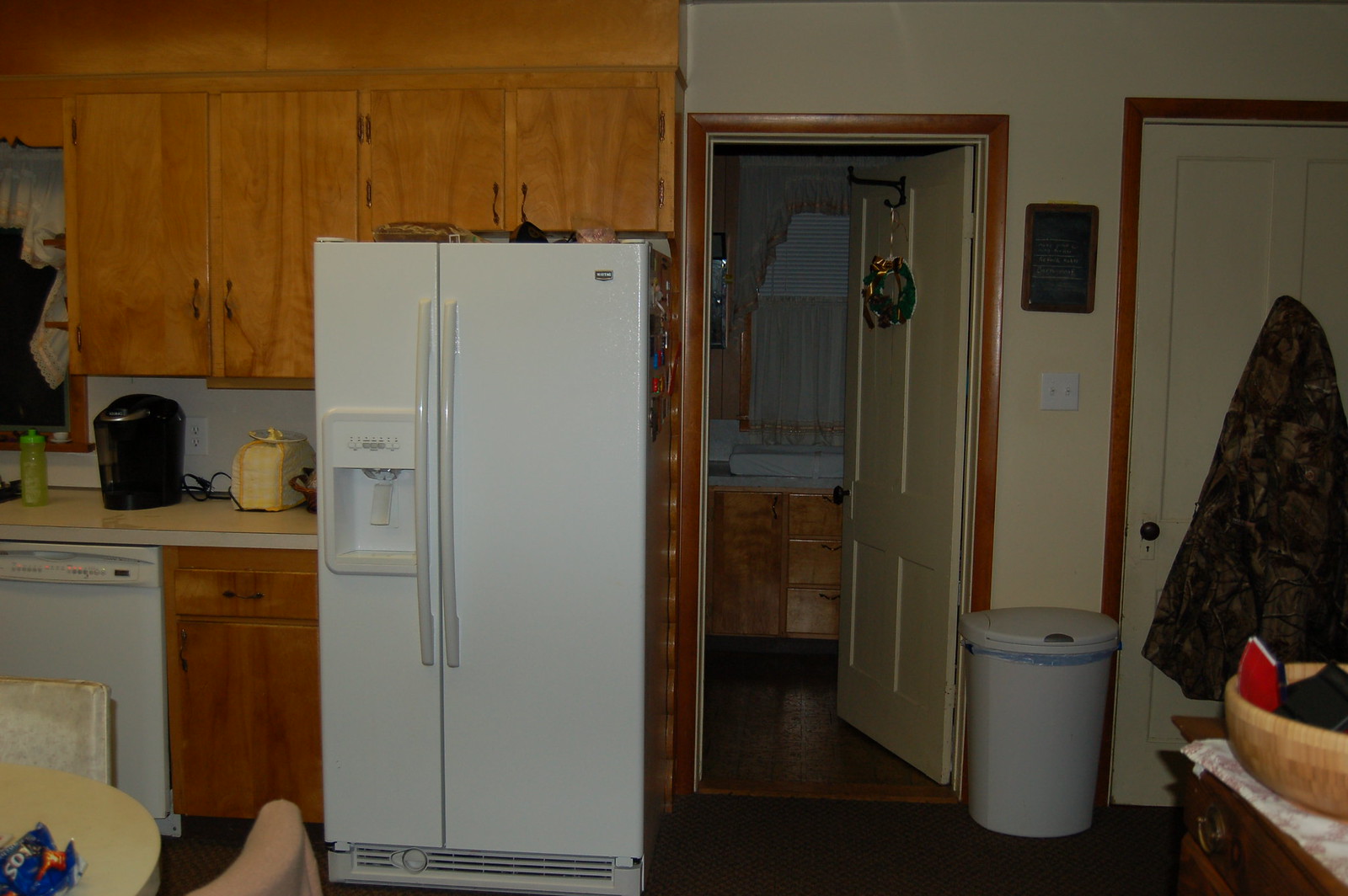This detailed photograph captures a cozy, possibly 1970s-style kitchen with a mix of modern touches. The kitchen features a cream-colored laminate countertop, light brown wooden cabinets, and a dual door white refrigerator equipped with an ice and water dispenser on the left door. To the left of the fridge, there is a white dishwasher, and further left on the countertop, a black Keurig coffee maker sits beside a lime green bottle—likely a kitchen cleaner or water bottle. Additionally, a yellow toaster is noted among the appliances on the counter.

Above the counter are more light brown wooden cabinets. In the foreground, the bottom left corner of the image displays part of a round Formica-style dining table with two chairs and a crumpled blue bag of Cool Ranch Doritos. 

To the right of the refrigerator, there is an open doorway leading to a bathroom, revealing a small window with a white curtain, a wooden countertop, and a line of drawers and cabinets of the same light brown wood. Between the bathroom doorway and another closed door to its right rests a gray trash can. A camouflage jacket is hung on the closed door, which also features a black handle. Adjacent to the jacket, there is a plaque with writing and a light switch. The bottom right corner of the image shows a dark brown dresser with a light brown wooden bowl containing various items.

Overall, the photograph captures a well-used, homey kitchen space with practical and aesthetic elements, including both vintage and modern accents.